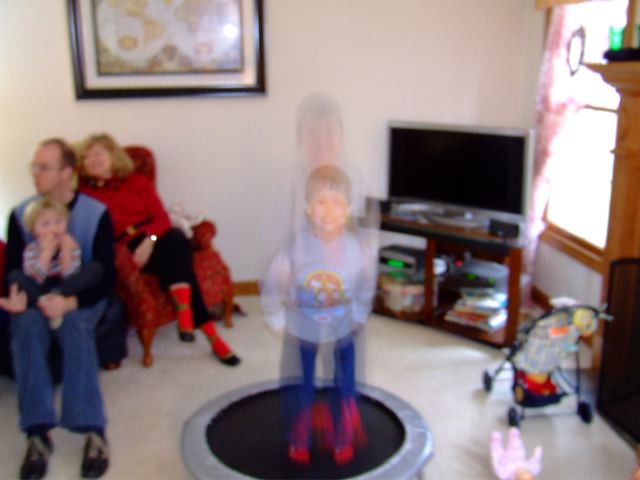In a bright, cozy TV room adorned with white walls and matching carpet, a little boy, about six or seven years old, leaps joyfully on a black mini trampoline with a silver-gray border. His motion creates a charming blur in the photograph, highlighting his playful energy. Dressed in a long-sleeved gray sweatshirt, blue pants, and vibrant red socks, he is the focal point of the scene. Behind him, sunlight filters through a window framed in dark wood with pink curtains, casting a warm glow into the room. In the corner, a wooden console cradles a smaller flat-screen TV.

To the boy's left, a woman sits in a red high-back upholstered chair featuring a subtle print. She is comfortably dressed in a long-sleeved red shirt, black pants, and red socks paired with black flats. Her blonde hair catches the light as she watches the boy with a gentle smile. Beside her, a man sits on a navy blue ottoman, cradling a little toddler in his arms. He is casually dressed in blue jeans, sturdy hiking shoes, a long-sleeved black shirt, and a light blue vest, completing the serene, familial atmosphere of the room.